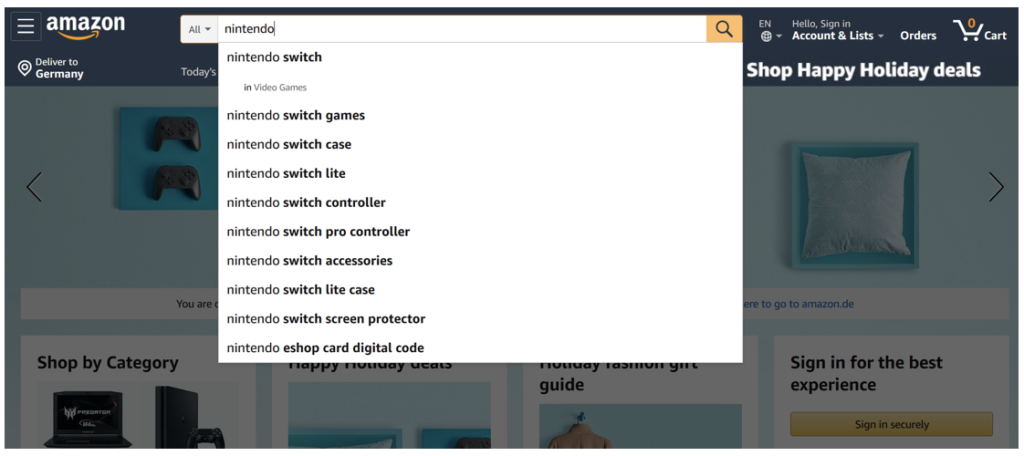**Descriptive Caption:**

The image captures a screenshot of an Amazon webpage with the search term "Nintendo" entered in the search bar. The search bar, which is white with black font, reveals a drop-down menu displaying various related search options such as "Nintendo Switch," "Nintendo Switch games," "Nintendo Switch case," among others. At the very top is the Amazon banner, featuring a black background with white text, which includes the "Amazon" logo on the left and a "Deliver to Germany" note underneath. On the right side of the banner, it indicates there are no items in the cart and promotes "Shop Happy Holiday Deals." Below the banner, the results for the "Nintendo" search occupy around four-fifths of the page. In the backdrop, somewhat faded, there are sections titled "Shop by Category" and "Sign in for the Best Experience," along with a few boxes displaying different product images.